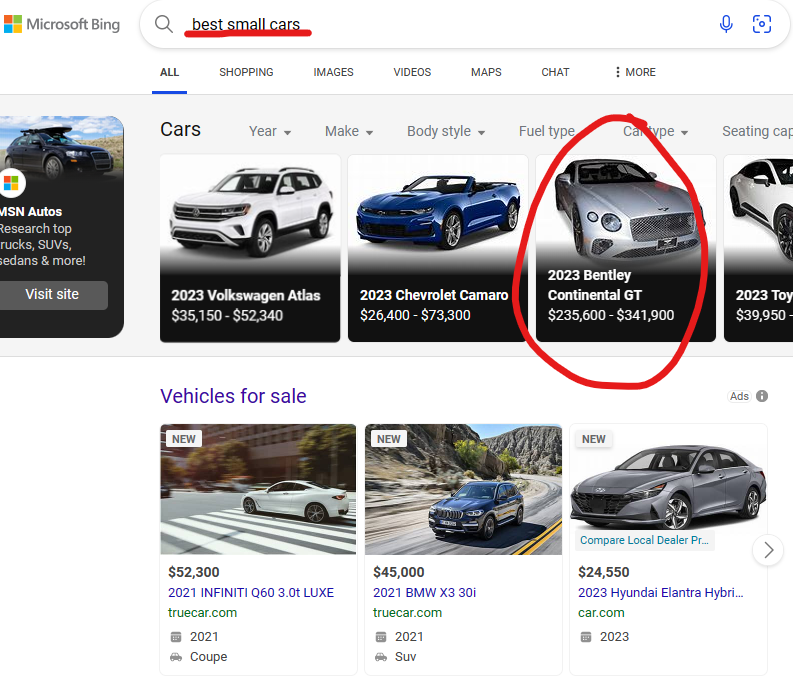Screenshot of Microsoft Bing search results for "best small cars"

In the upper left-hand corner, a small, square Microsoft logo displays the red, green, blue, and yellow colors. To the right of the logo, "Microsoft Bing" is written in light black font. 

Below this, an oval search bar stretches horizontally across the screen with a gray magnifying glass icon on its left side. To the right of the search bar, the words "best small cars" are displayed in black and underlined with a thick red line. 

Dropping down, a menu line features the word "ALL" in bold, uppercase gray letters and underlined in blue. Following "ALL" from left to right, the menu includes "Shopping," "Images," "Videos," "Maps," "Chat," and an icon of three blue dots for "More."

Beneath the menu, the left side of the screen partially shows an ad for MSN Autos, which is cut off. Next to the ad, the word "Cars" appears in black text. Below "Cars," gray tabs labeled "Year," "Make," "Body Style," "Fuel Type," and "Car Type" span horizontally. Below these tabs, the partially visible word "Seating" appears with a cutoff "CAP."

Further down, several photographs of cars are displayed. They include images of a 2023 Volkswagen Atlas, a 2023 Chevrolet Camaro, and a 2023 Bentley Continental GT. The Bentley image is circled with a hand-drawn red circle. Part of a fourth car image is visible with the text "2023 TOY" partially showing.

About five lines below the initial set of photographs, three more car photographs are displayed along with their prices.